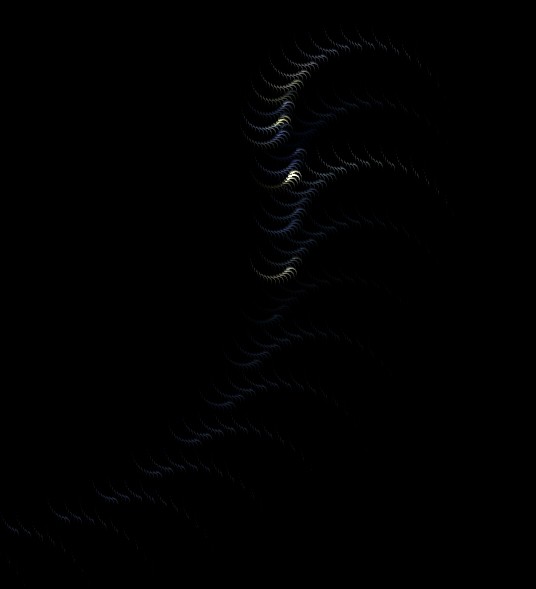The image depicts an almost completely black background with a series of peculiar white, wispy structures visible primarily at the top right and extending vertically downwards across the page. These structures appear organized in four repeating rows, starting off dark and gradually becoming lighter, interspersed with patches of yellow. Upon zooming in, it becomes evident that these lines continue all the way to the bottom, albeit most of them lack the yellow ends—specifically, three lines feature the yellow sections while seven or eight do not. The wispy formations give an impression reminiscent of dragon skin, with the background's blackness emphasizing their intricate design. Lower on the left side, smaller waves or spikes arise, gradually increasing in height and culminating at the top in tan or gold hues, contributing to the overall mystique. The surreal, almost monstrous ambiance suggests it could be a scene straight out of a video game or a movie, evoking imaginations of fantastical creatures.